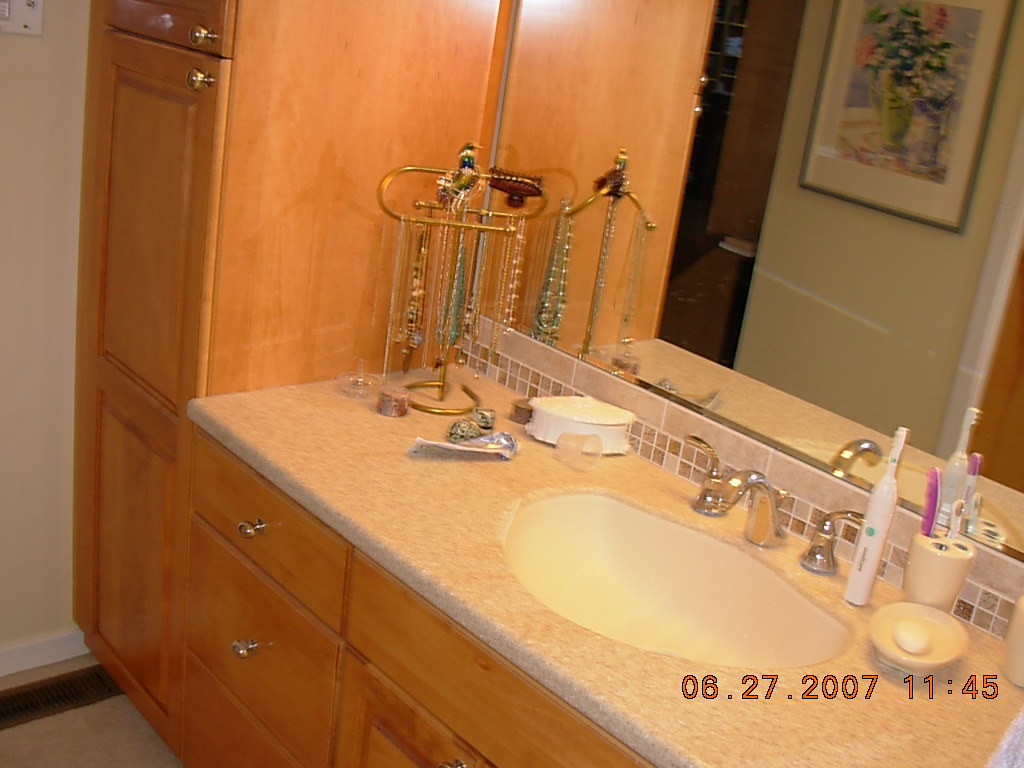In this indoor photograph of a bathroom vanity, the focal point is a well-organized and chic sink setup. On the left-hand side, a tall wooden cabinet extends upward, partially cropped from the image, adding a touch of natural warmth to the space. Adjacent to the cabinet is a large mirror that reflects part of the opposite wall, which is adorned with a framed illustration of a vase filled with flowers, injecting a bit of art and color into the setting.

The sink, prominently placed in front of the mirror, features an irregularly shaped oval basin, pristine white on the inside, complemented by sleek chrome fixtures that exude contemporary elegance. To the right of the fixtures, an electric toothbrush stands upright, flanked by a cream-colored ceramic toothbrush holder and a matching soap dish, which cradles a small bar of white soap, creating a harmonized look.

The countertop, with its brown and white granite appearance, adds a sophisticated touch to the vanity area. On this surface, to the left of the sink, a metal necklace stand displays an assortment of beaded necklaces, possibly infusing a personal or decorative element to the setup. A mostly flattened tube of toothpaste lies nearby, a small but essential detail that hints at the daily use of this space.

Beneath the sink, two wooden drawers with chrome handles offer practical storage solutions while maintaining the cohesive aesthetic of the bathroom. The overall composition of the photograph suggests a blend of functionality and style, making it a visually pleasant and utilitarian space.